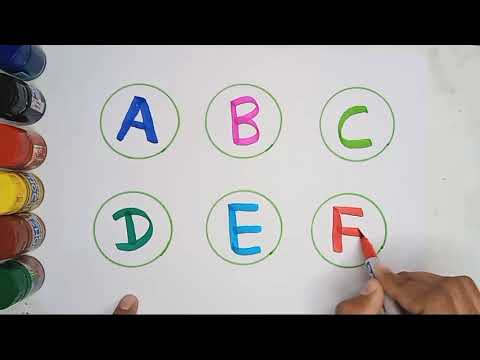In this photograph, a person with light brown skin is seen drawing on a white piece of paper. The image is bordered with vertical black strips at the top and bottom. The person’s left hand is partially visible with a finger resting on the paper, while their right hand, holding a red marker, is actively drawing the letter "F," which is enclosed in a green circle. Centered on the paper are letters "A" through "F," each circled in various colors—specifically, a blue "A," a pink "B," a green "C," a blue-green "D," a teal "E," and the ongoing red "F." To the left of the paper, there is a row of colorful bottles, possibly containing ink or paint, arranged vertically. The colors of these bottles from top to bottom are dark blue, black, orange, yellow, red, and green. The overall scene suggests a creative or educational activity.